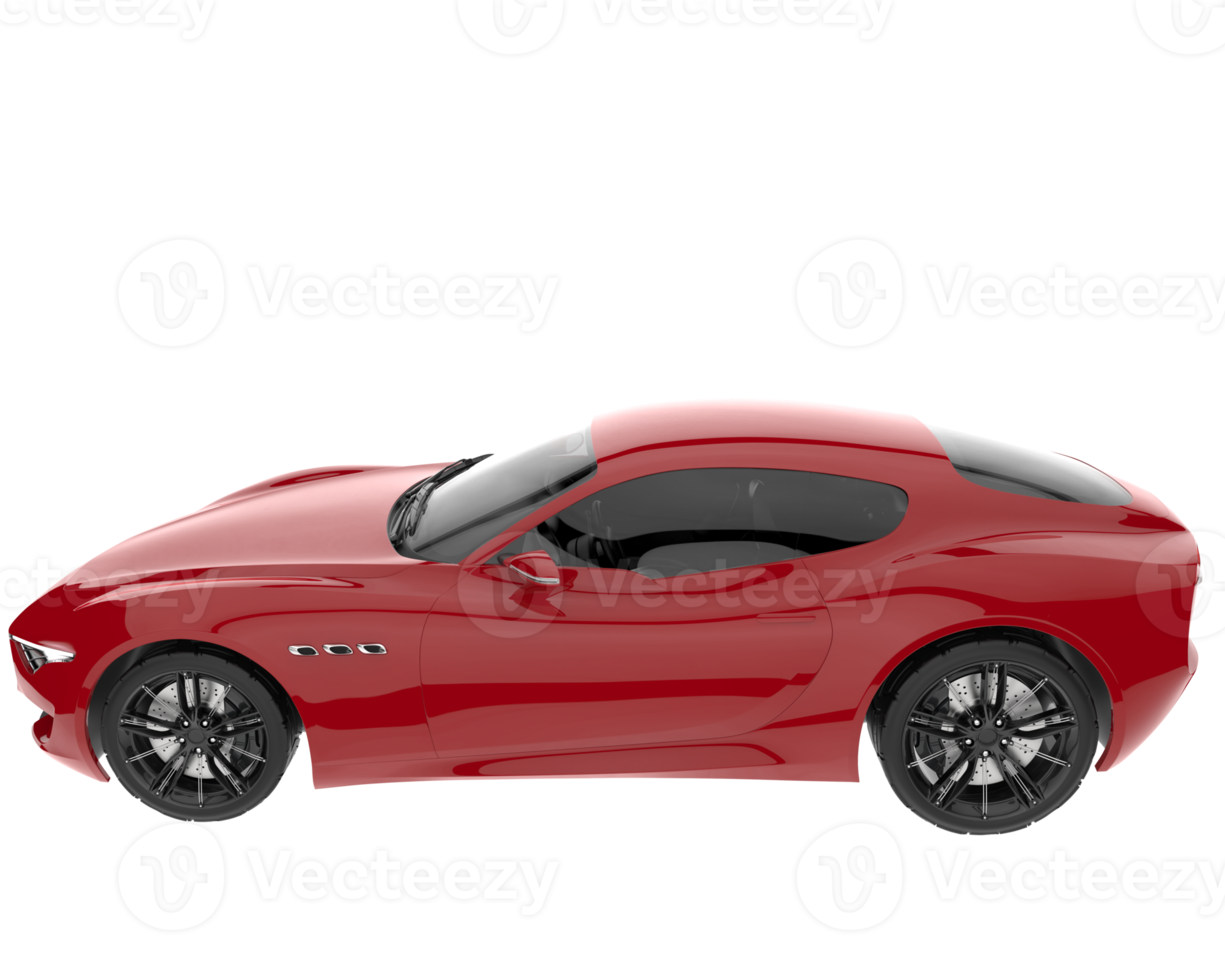This detailed image portrays a sleek, red coupe reminiscent of the design aesthetics of a Mazda Miata or Porsche Boxster. The car boasts a striking, compact form with an extended front and a squat rear, perfectly capturing the essence of a two-seater sports car. Its large black wheels add to its sporty appearance, and the interior is equally stylish with an all-black finish. The image is overlaid with a light gray watermark of the old Vine logo and the text "Vecteezy," which repeats in four horizontal lines across the black background, subtly imparting a textured look.